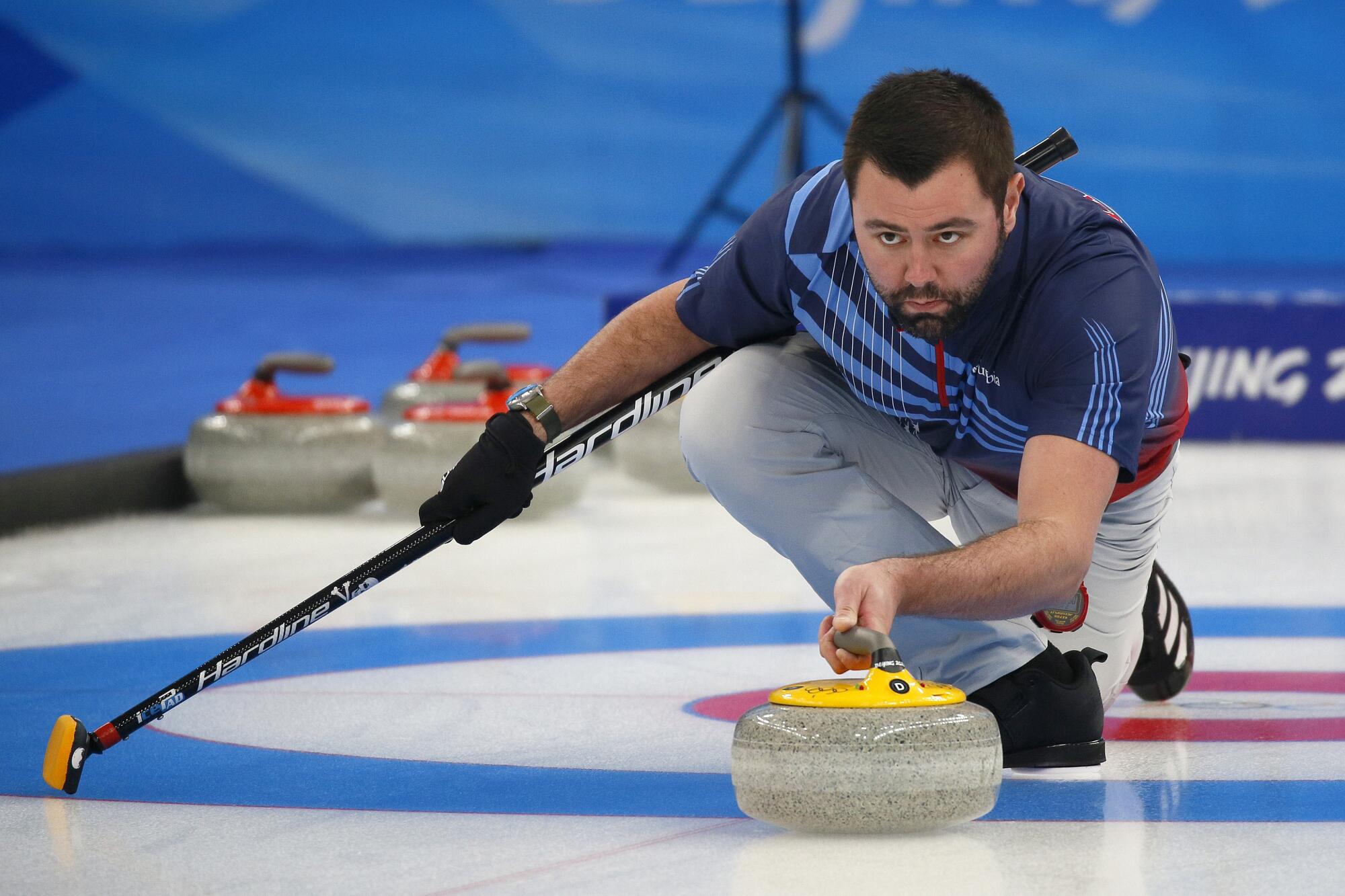This high-resolution, horizontal color photograph captures a detailed scene from a curling match featuring a Caucasian man with a beard and short hair. He is wearing white khakis, black shoes, and a dark blue uniform shirt with light blue stripes. Positioned on the right side of the image, the man is crouched with his right knee bent on the ice and his left foot planted, exuding a sense of concentration and strategy. His right hand, gloved in black and adorned with a watch, grips a curling stick that has a black shaft with a soft, orange broom-like pad on the end, inscribed with the text "hardling."

In his left hand, he firmly holds a smooth, glossy curling stone made of granite, which is silver with a yellow handle. His poised stance and focused expression imply he is meticulously aiming to push the curling stone forward. Behind him, on the left side of the image, three additional curling stones with red tops can be seen, along with a tripod set up in the middle background. The entire scene vividly portrays the intensity and precision required in the sport of curling.